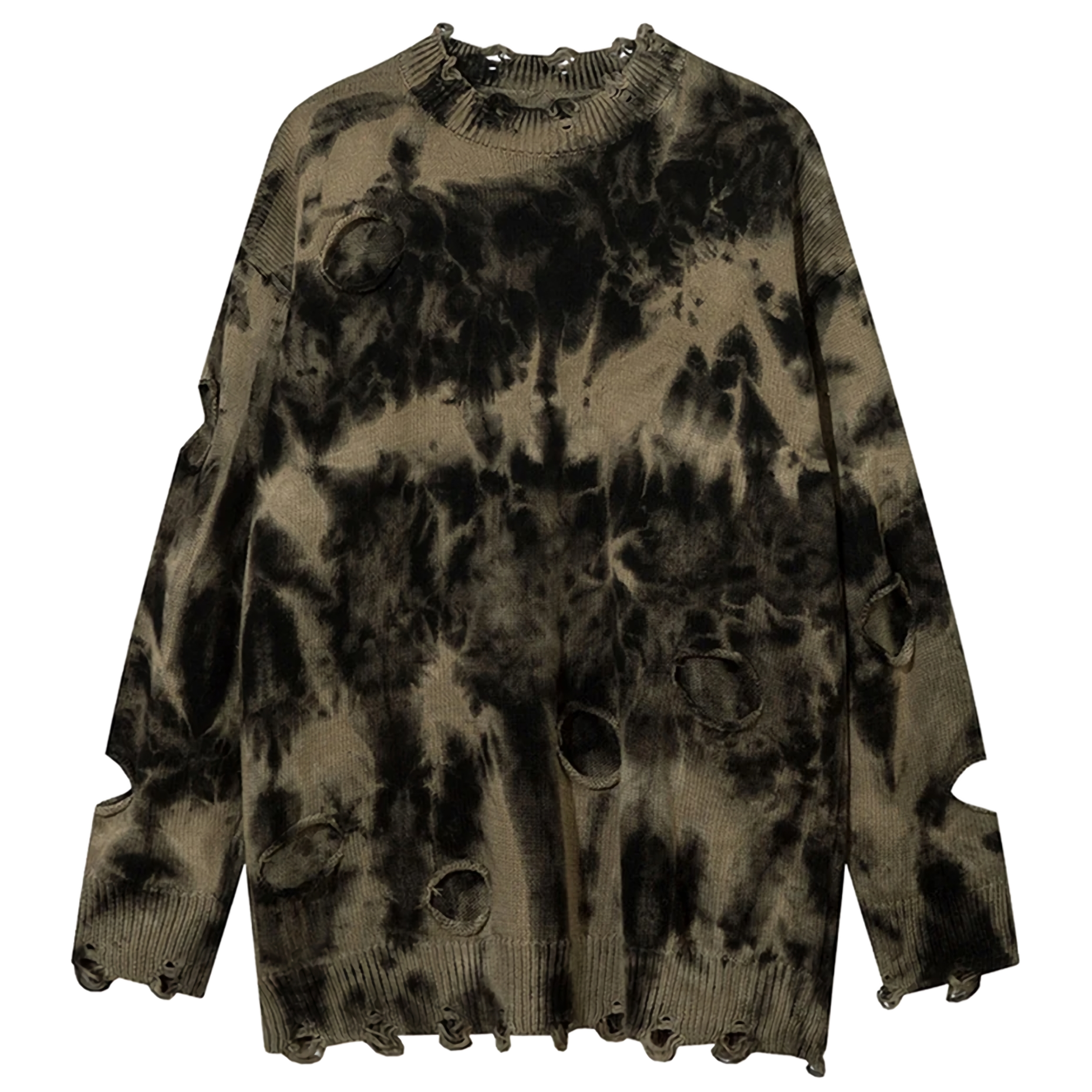This image features a long-sleeve, distressed knitwear top, showcasing a grungy and fashionable aesthetic. The sweater, made of wool, is primarily canvas brown with dark black and gray blotches that create a tie-dye effect. Its collar, sleeves, and hem are ribbed but heavily torn and weathered, enhancing its distressed look. Numerous holes, about an inch long, are sporadically placed along the front, sleeves, and waistband, contributing to its tattered appearance. The neck area, along with the ends of the sleeves, displays additional distressing with several holes. The garment, possibly intended for a male and evocative of streetwear fashion, lies flat against a stark white background, suggesting it might be showcased on an online clothing catalog.